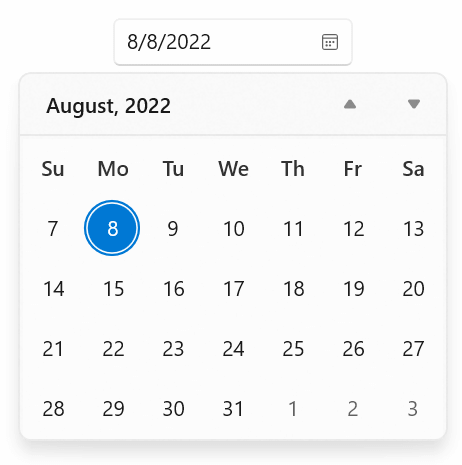Below is the cleaned-up and detailed caption for the image described:

---

The image showcases a detailed view of a calendar feature from an application or website. The overall background is white. At the top of the screen, there is a centered, semi-designated search bar area, outlined with a thin gray line. This area contains a calendar icon on the right and displays the date "8/8/2022" (August 8th, 2022) on the left.

The search bar area is centered horizontally, occupying approximately half the screen's width, with equal blank white spaces on its left and right sides.

Beneath this central search area is the main calendar display, which is similarly outlined with a thin gray line. A thin gray line horizontally divides the calendar, with the portion above the line having a light gray background and bold black text that reads "August, 2022." To the right of the text are two solid gray triangles – an upward-pointing one above a downward-pointing one, likely for navigating between months.

The main calendar grid rests below this heading, set against a white background. The days of the week are labeled in bold: "SU" for Sunday, "MO" for Monday, "TU" for Tuesday, "WE" for Wednesday, "TH" for Thursday, "FR" for Friday, and "SA" for Saturday.

The calendar starts with Sunday, August 7th, since only the latter part of the month is displayed, focusing on operating around the chosen date of August 8th. This specific date, August 8th (Monday), is distinctly highlighted with a blue circle that includes a thinner white border inside and an outer blue border, resembling a target.

The subsequent days are arranged in a weekly format:
- First row: August 7th to August 13th
- Second row: August 14th to August 20th
- Third row: August 21st to August 27th
- Fourth row: August 28th to September 3rd, including the first three days of the following month

A subtle shadow effect outlines the left, right, and bottom edges of the calendar for a slight elevation effect, although this shadowing effect does not extend across the top of the calendar.

---